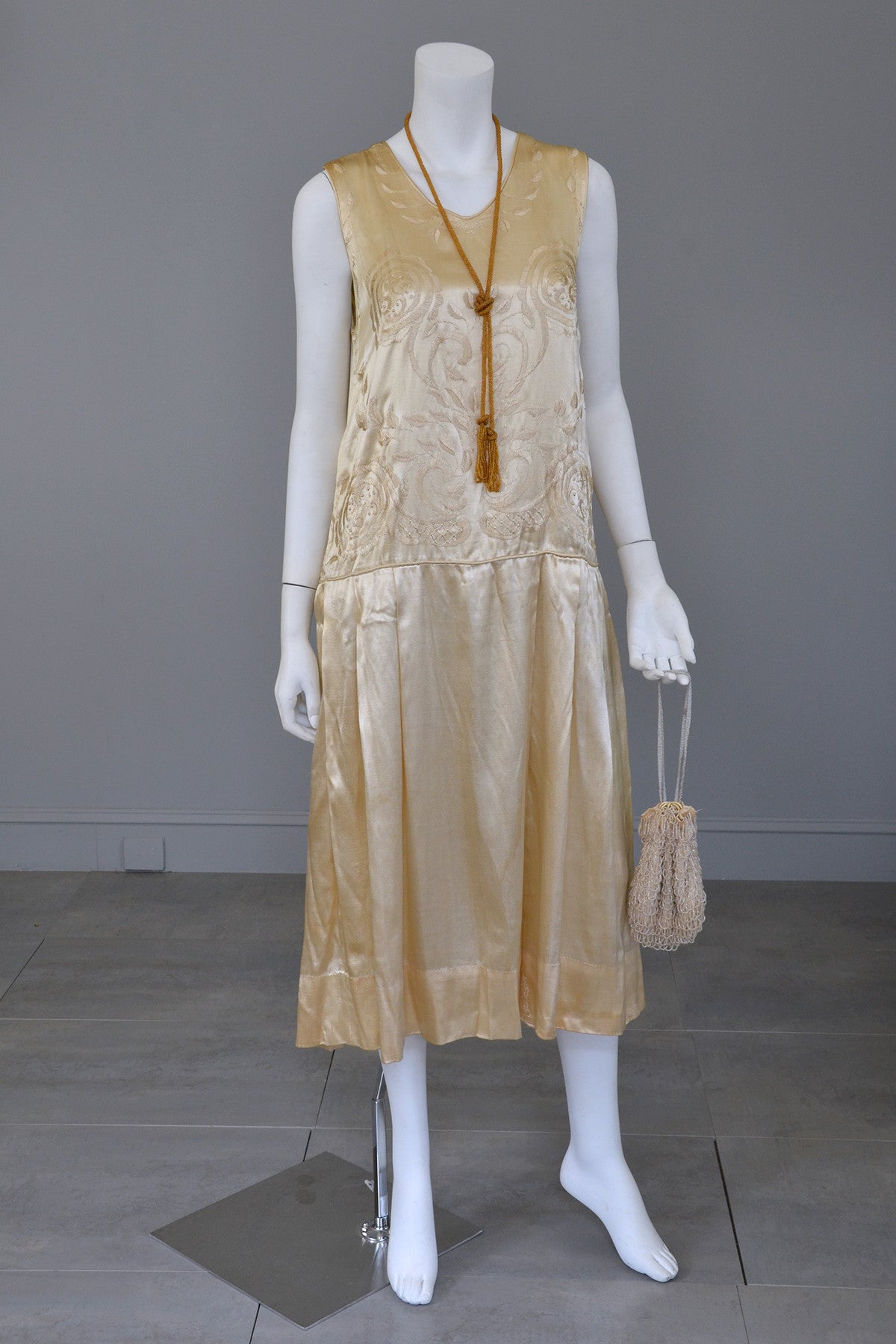This image features a headless female mannequin situated on a grayish rectangular tile floor. The background wall is a solid off-white color. The mannequin, which has a traditional white cream skin tone, is dressed in a light gold-colored, sleeveless one-piece dress that extends to mid-calf, featuring a light floral print embossed in the collar area on the chest. The dress has a silky and shiny appearance, reminiscent of vintage styles, possibly from the ragtime era. Accessories include a long gold-corded necklace, which dangles from halfway down the neck, and an older-style small gold handbag held in the mannequin's left hand. A darker-colored square tile, different in size from the rest of the flooring, is placed next to the mannequin's foot, adding to the display scene, which appears to be set up in a store.